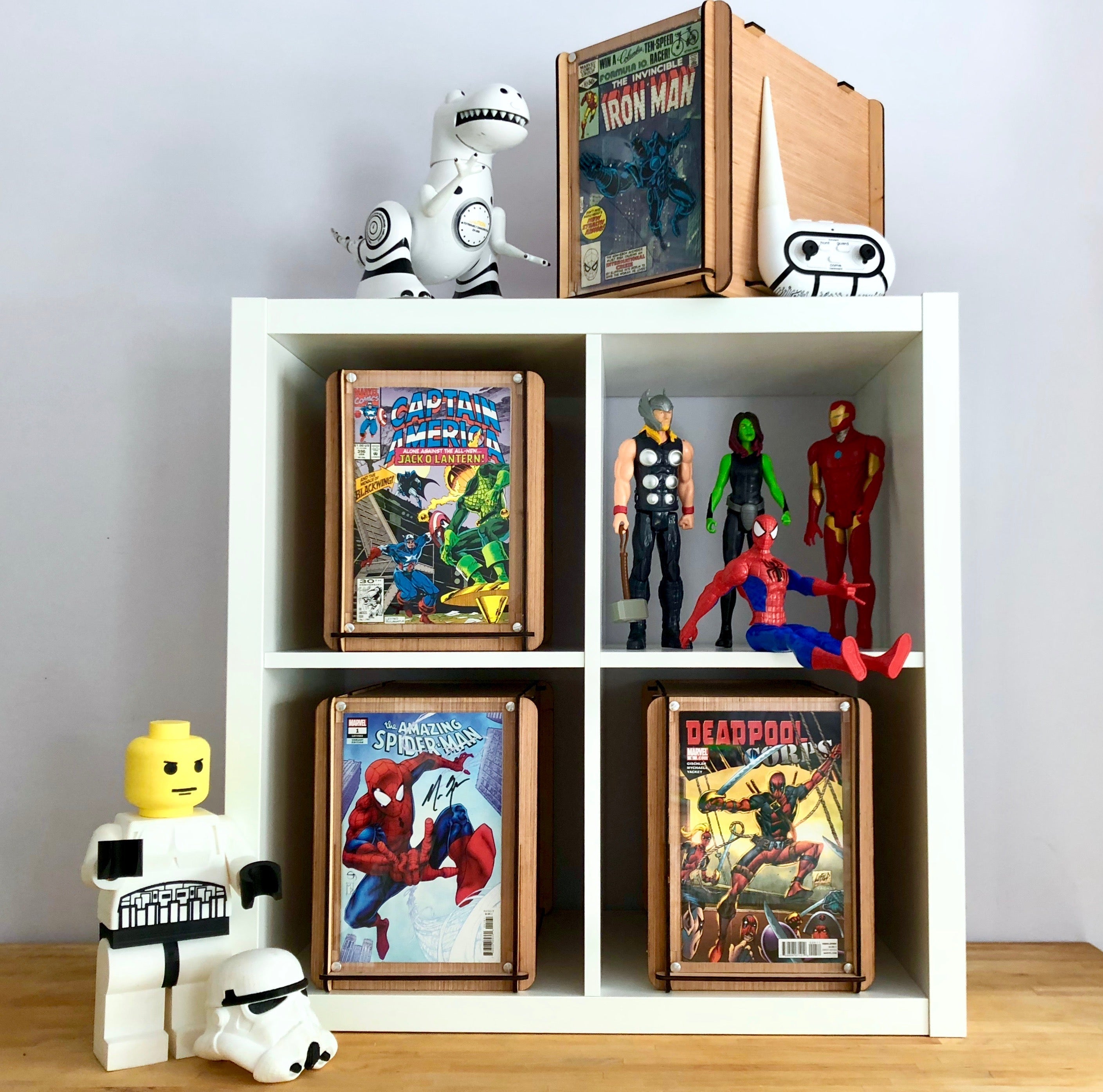This detailed image depicts a white four-section display shelf measuring approximately 24 by 24 inches, situated against a gray wall on a wooden floor. The shelving unit is divided by a central separator, creating four equal squares, each containing an array of collectibles, notably centered around superhero themes.

Starting at the top, placed on the shelving unit's surface, there is a clock embedded in a T-Rex toy that resembles the character from Toy Story. This mechanical dinosaur is predominantly white, black, and gray. Adjacent to the T-Rex is a larger wooden box showcasing "The Invincible Iron Man" comic. Right next to this is a smaller controller with a pronounced spire, two black toggles, and white buttons marked with black text, though the text is too small to decipher clearly.

Moving to the individual sections of the shelving unit:

- **Top Left Section**: Features a balsa wood box displaying a “Captain America” comic with illustrative blue and white stripes. Inside the box, there is a visibly green antagonist engaged in combat with Captain America.
- **Top Right Section**: Houses an array of figurines including Thor with his hammer and winged helmet, She-Hulk dressed in a sleeveless black suit with green skin and brown hair, Iron Man donning his iconic red and gold armor, and Spider-Man posed with his hand extended in a rock-and-roll sign and feet dangling over the ledge. 
- **Bottom Left Section**: Contains “The Amazing Spider-Man” comic displayed on the shelf, with a dynamic image of Spider-Man leaping towards the front.
- **Bottom Right Section**: Features a boxed “Deadpool Corps” comic book, depicted with Deadpool holding a sword. In front of the comic, a larger-than-life Lego figurine fashioned as a Star Wars stormtrooper is set up, with his helmet removed revealing a yellow head above the white armor suit.

This intricate amalgamation of comics and figurines highlights a deep passion for superhero lore, meticulously arranged to create a visually engaging display.